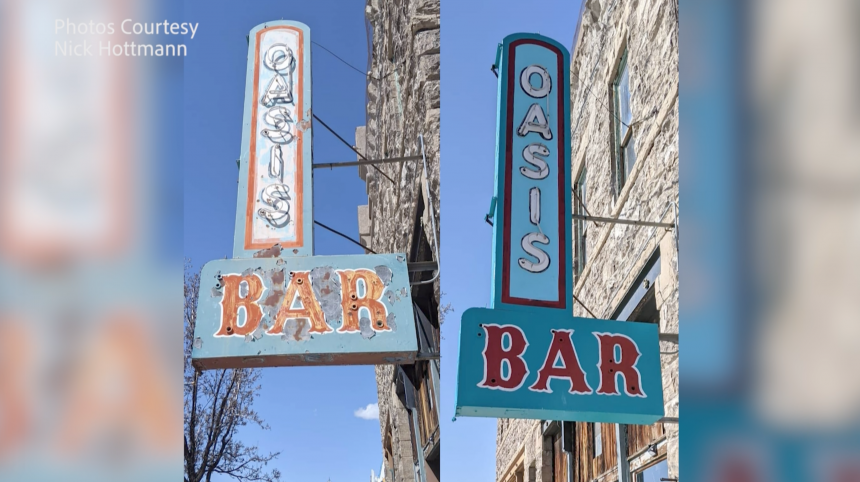This image is a side-by-side comparison of two photographs showcasing an overhead sign for the Oasis Bar attached to a stone building. The left photograph displays the sign in its original, worn state, with rust, faded colors, and overall dirtiness. The letters "OASIS" are aligned vertically in orangish, faded paint, and "BAR" stretches horizontally in the same worn-out coloring. Below the sign, a tree can be seen growing next to the rusted section.

In contrast, the right photograph depicts the refurbished sign, boasting a vibrant transformation. The background is freshly painted in blue, with "OASIS" in bold white letters standing out prominently in a vertical arrangement. Meanwhile, "BAR" appears horizontally in striking red letters. The signage, which extends outward and is bolted to the building, appears much cleaner and updated, with the neon elements brightly illuminated. The stone building retains its original character, with wooden-bordered windows visible in the background.